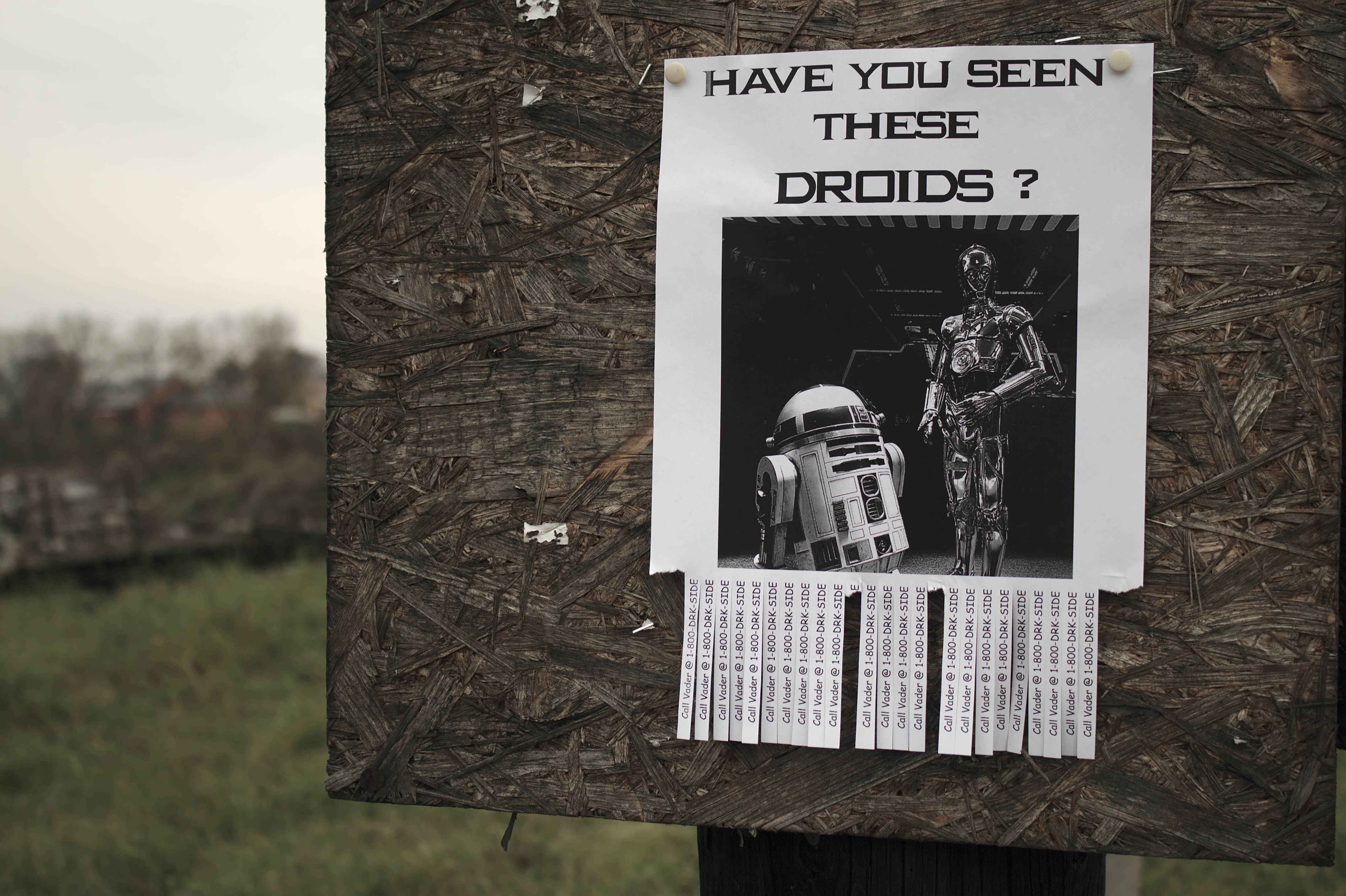This photograph captures a comedic "missing persons" flyer clearly spoofing Star Wars, adeptly situated on a brown particle board mounted on a large wooden post. The flyer, printed on white paper with a black font, prominently reads "Have you seen these droids?" at the top. Beneath this headline, black-and-white images of the iconic Star Wars characters R2-D2 and C-3PO are juxtaposed, with R2-D2 on the left and C-3PO on the right. Below the images, tear-off tabs display the humorous message, "Call Vader at 1-800-DARKSIDE," inviting those who spot the droids to reach out. The background reveals a blend of greenery with grass at the bottom and taller trees in the middle, and a muted gray sky, affirming that the photo was taken outdoors during the daytime. The flyer is affixed to the particle board using staples and push pins, amidst remnants of other scattered papers and staples.